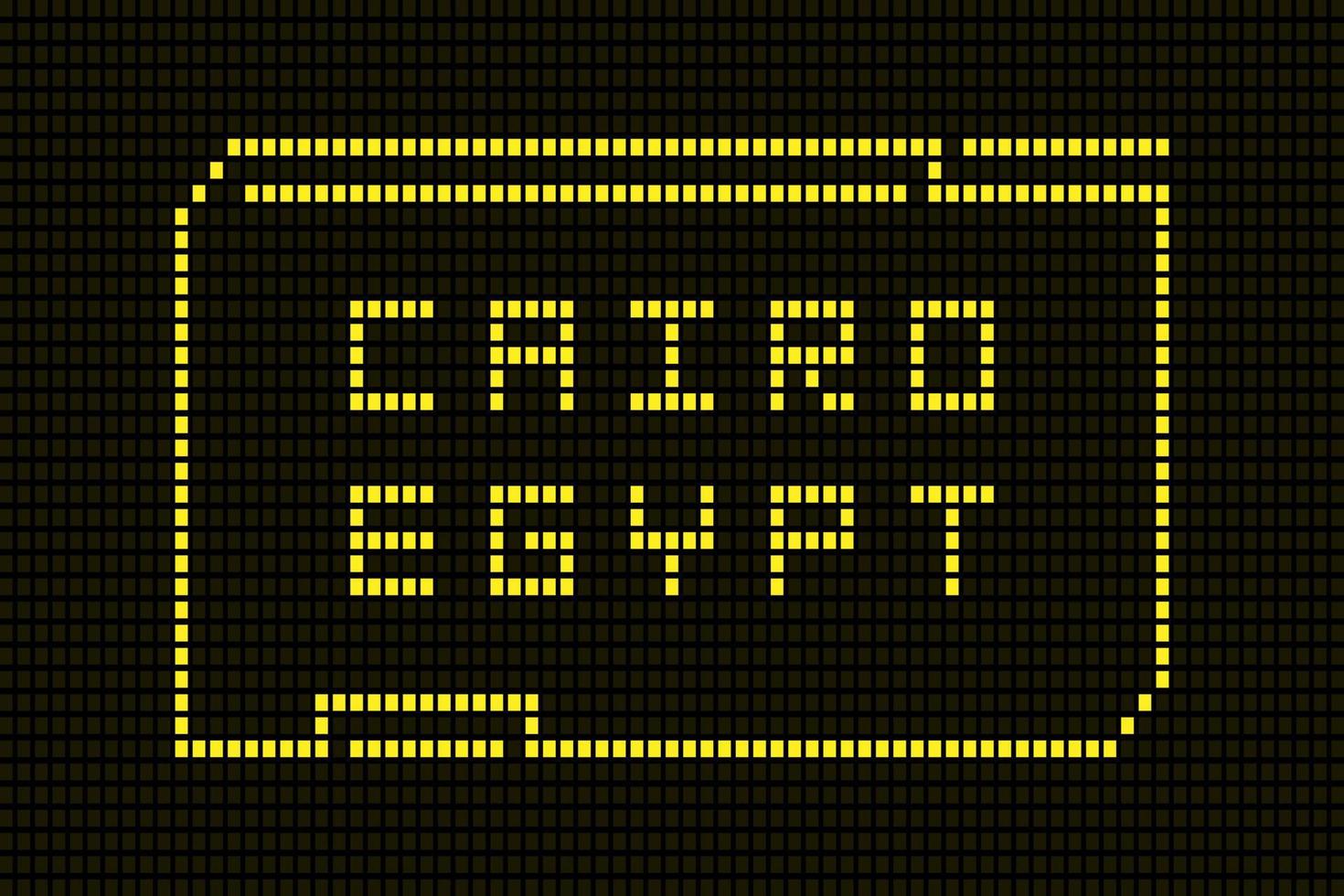This image resembles a pixelated digital artwork composed of numerous tiny square blocks arranged in a meticulously aligned square grid. The predominant background is formed by small black squares. In the middle of the grid, there is a prominent rectangular block made out of closely lined yellow squares. Within this yellow rectangle, the words "Cairo, Egypt" are symmetrically spelled out, also in yellow pixels, matching the color of the rectangular border. This creates a striking contrast against the black background, emphasizing the textual content. The overall design is reminiscent of a digital sign with "Cairo, Egypt" in bright yellow lettering, bordered by a yellow rectangular frame, all set against a black pixelated canvas.